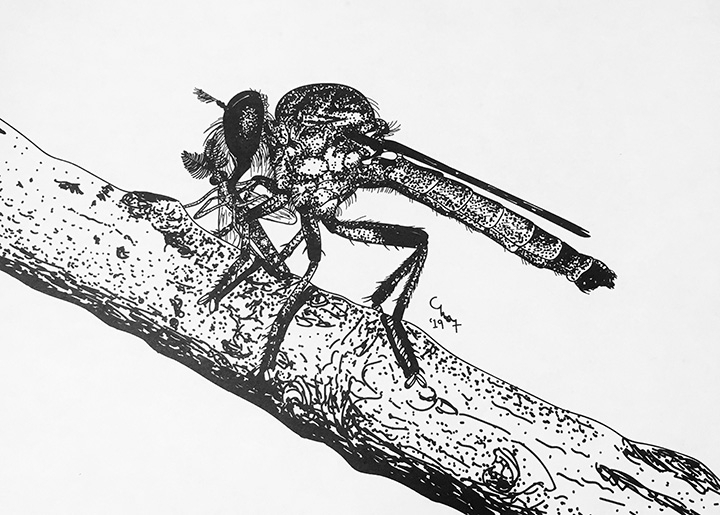This black and white sketch rendering depicts a detailed dragonfly perched on a textured branch. The branch, etched with intricate lines and crevices, diagonally spans the foreground from the top left to the bottom right against a gray background. The dragonfly, identified by its long, dark-shaded legs and distinctive bulging eyes, features a spotted black and white body with its wings folded back along its torso. The drawing is signed "Chalks 19" near the dragonfly's legs, and it appears to be holding another insect, possibly as prey, in its mouth. Shadows and detailed shading add a sense of depth and realism to the illustration.